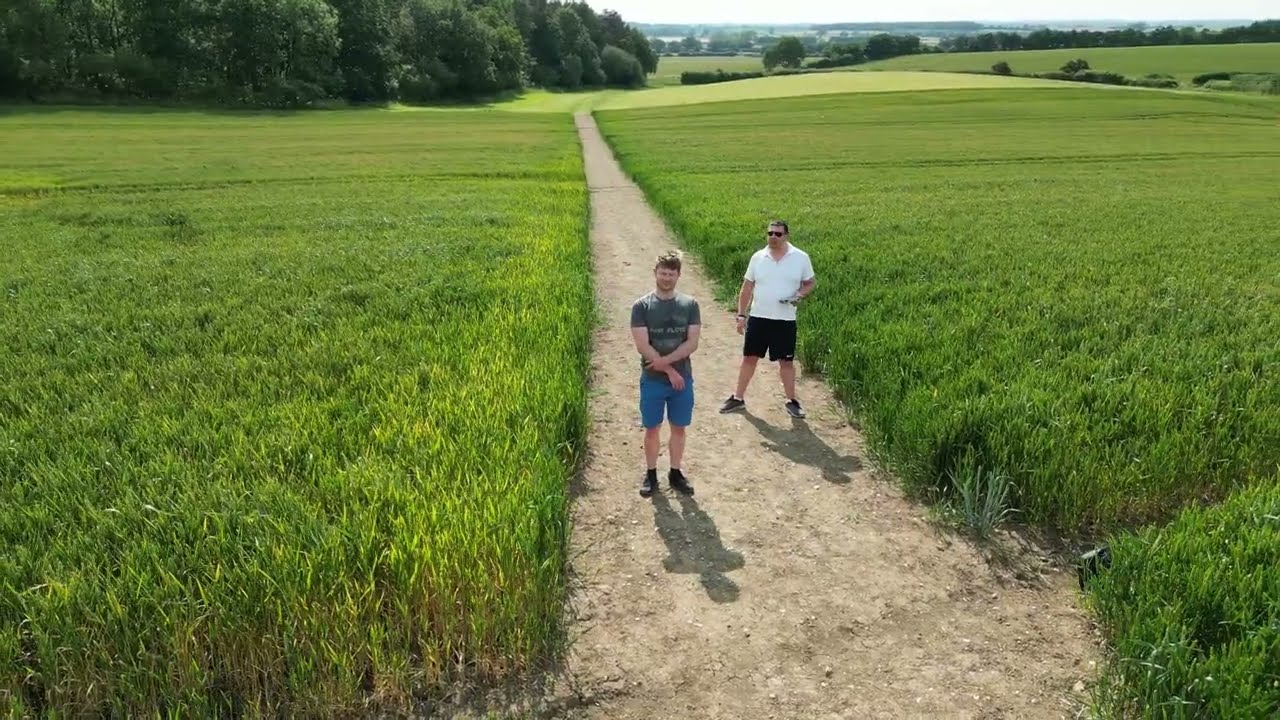The image is a slightly high-angle shot, likely taken from an 8 to 10 feet height, possibly by a drone. It captures a neatly maintained dirt path running through a vast farmland or grassland area, characterized by dry, cracked soil and even rocky patches. The path is flanked by uniform, tall green grasses that resemble still-growing wheat or some other dense vegetation. This rural setting appears prosperous and meticulously cared for, with the greenery extending for miles, dotted occasionally by clusters of thick trees forming small forested areas.

In the foreground, two men stand on the path. On the left is a young man, seemingly in his 20s, wearing a grey t-shirt, blue shorts, and black trainers. He has light brown hair, his arms crossed in front of him, and is looking towards the drone. To his right stands an older, slightly balding man in a white t-shirt, black pants, and sunglasses. He stands with his legs apart and his right arm holding something close to his body while his left arm hangs by his side, also looking in the direction of the camera.

Beyond the men, the fields stretch into the distance over slightly sloping hills, creating a picturesque, pastoral scene that is both clean and fresh. In the background, a forested area can be seen, and far off on the horizon, structures suggesting a town or city are faintly visible. The bright, sunny day enhances the vibrant greens and overall serene atmosphere of this rural landscape.